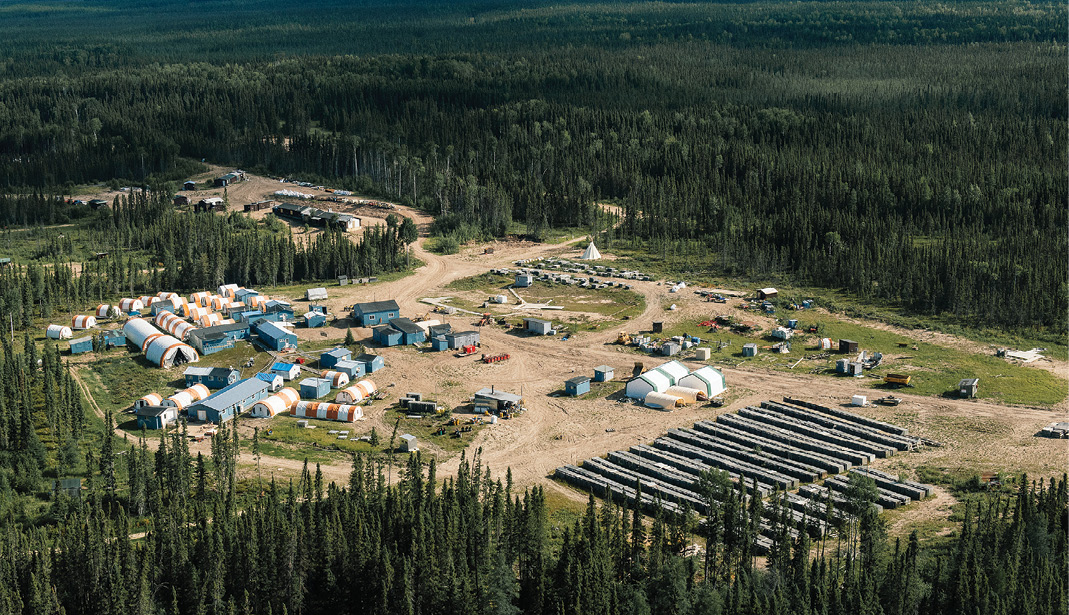An aerial view captures a bustling encampment deep within a forest. The image reveals an intricate setup of white tents with orange stripes and several blue buildings with matching roofs, all nestled in a cleared section surrounded by dense, leafy green trees. In the top distance, a sea of greenery extends, while the middle of the image features a mix of trees, open spaces, and dirt pathways. Visible is a gravel road that curves through the site, leading to various structures that range from large blue buildings to smaller, half-circle tent-like formations and tiny white constructions. A teepee stands near the edge of the compound, which is bordered by more forest and crisscrossed by gravel lanes extending out of sight. The lower portion of the image shows rows of unidentified black and white objects, alongside more tall, skinny trees that encapsulate the bottom edge. Despite the absence of visible individuals, the encampment exudes a sense of organized activity and purpose amidst the secluded woodland.